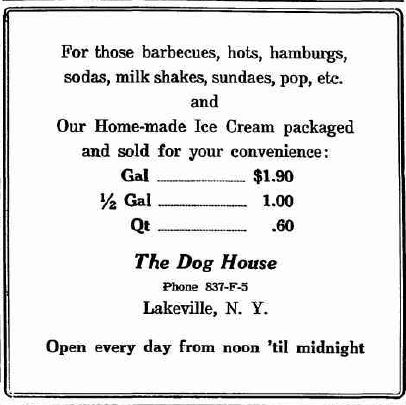The image portrays a square-shaped, black-and-white advertisement, reminiscent of an old newspaper snippet. The ad features a plain white background, enclosed with black double borders. Centrally positioned text reads: "For those barbecues: hots, hamburgs, sodas, milkshakes, sundaes, pop, etc., and our homemade ice cream packaged and sold for your convenience." Below this, it lists three purchasing options for the ice cream in bold black text: a gallon for $1.90, a half gallon for $1.00, and a quart for $0.60. At the bottom of the ad, the name "The Dog House" is prominently displayed, followed by a phone number (837-F5), the location "Lakeville, New York," and the operating hours "Open every day from noon till midnight."